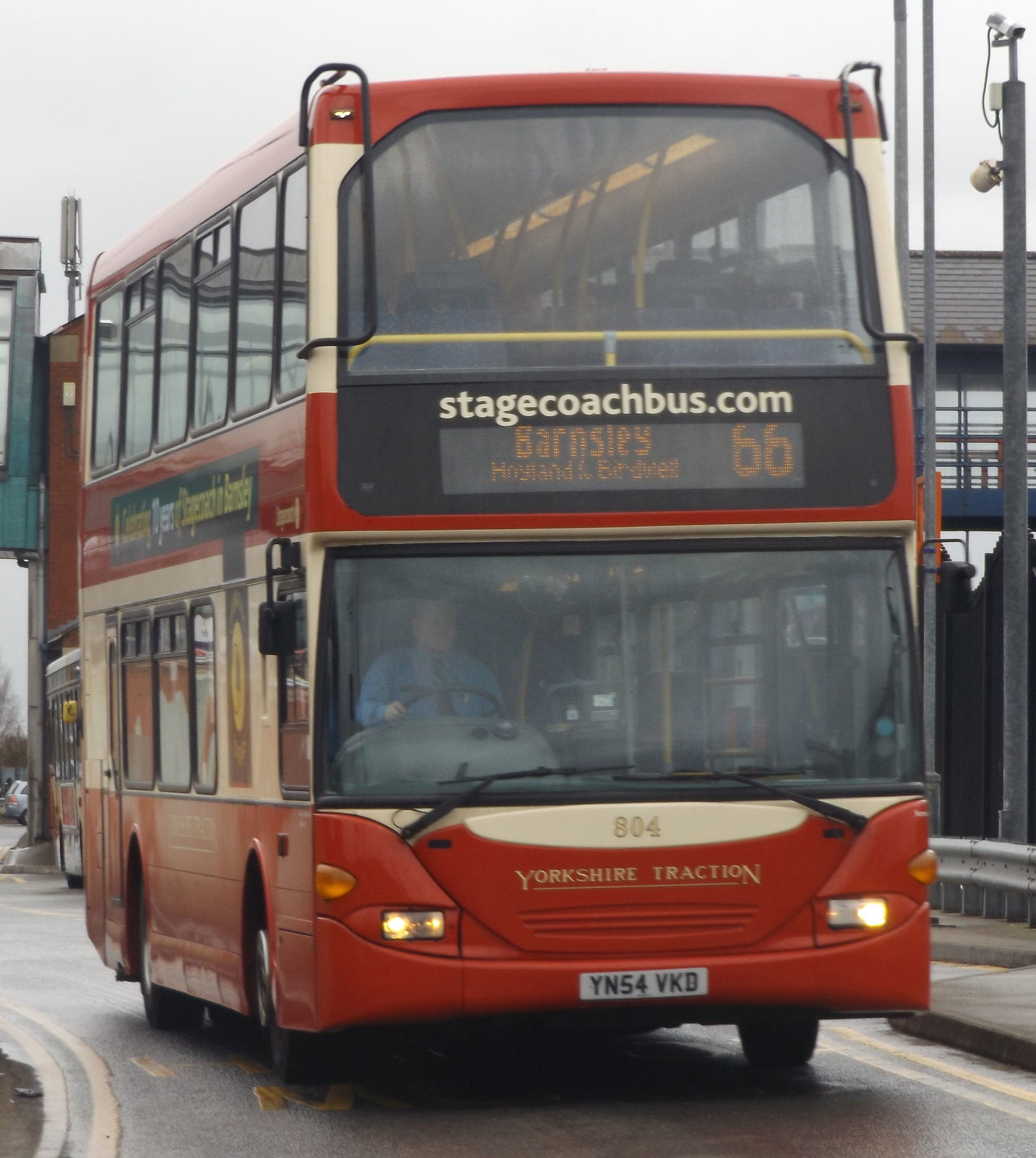The image depicts a large, red, double-decker bus traveling down the road against a light blue-gray sky backdrop. The bus is seen from a front side angle, prominently showcasing its clean, red exterior with white trim and gold lettering. A tan banner spans the middle between the two stories of the bus, displaying "Stagecoachbus.com." Below, an electronic sign reads "Barnsley," while adjacent to it is the number 66. Text on the bottom line of the electronic sign is partially legible, mentioning Barnsley, Hoyland, and Birdwell. The bus features an upper deck front window and a lower deck window, with gold lettering of the bus number 804 conspicuously displayed below. In gold letters, the name "Yorkshire Traction" is also visible on the red front. The bus's white license plate reads YN54BKD. A male driver, dressed in a blue shirt and tie, is seated on the left side of the bus, adhering to the driving position on this particular road. Behind the bus, a building is somewhat obscured from view.